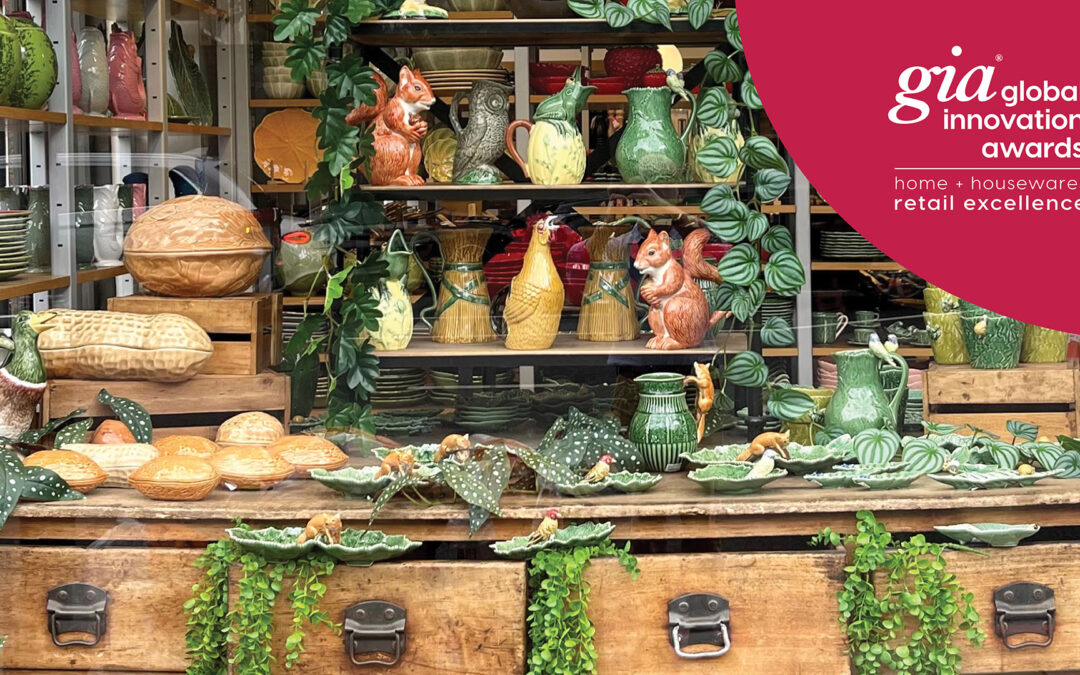The photo depicts a close-up of a stylish, wooden shelving unit, likely from a homeware store or interior decor setting, adorned with a variety of detailed and whimsical decorations. Open wooden drawers spill out lush artificial greenery, adorned with ceramic figurines—a bird perched on a leaf in one, and a fox on another. Atop the shelves lies an array of natural-themed figurines, predominantly in green and brown hues, including ceramic peanuts and walnuts, squirrels, and owls. The display also features green and yellow vases, plates, and pitchers, contributing to the overall earthy aesthetic. The motif emphasizes green with brown accents, with a focus on animals and nature. Additionally, a red circular emblem on the right side signifies an award from the GIA Global Innovation Awards for Home and Houseware Retail Excellence. The shelving unit itself is brown with silver handles, enhancing the natural yet sophisticated vibe of the overall arrangement.